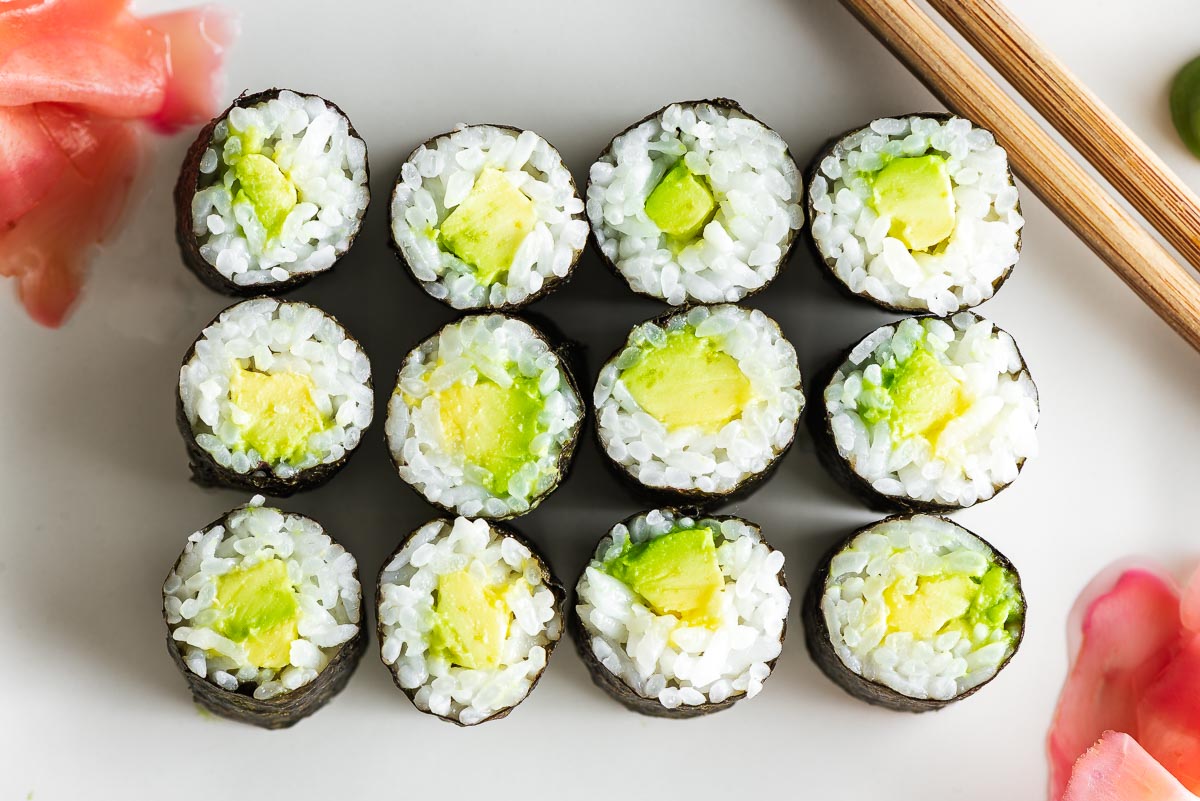The photograph showcases a neatly arranged set of 12 small sushi rolls, presented in three rows and four columns, placed on a white surface that appears to be a plate. Each roll consists of white rice and a green filling that seems to be avocado, encased in a thin layer of seaweed. To the top left and bottom left of the image, there are small piles of thinly-sliced, rosy-colored ginger. Partially visible wooden chopsticks extend into the frame from the top right corner. The image is captured from a top-down perspective under dim lighting, emphasizing the shadows and details of the sushi and garnishes.